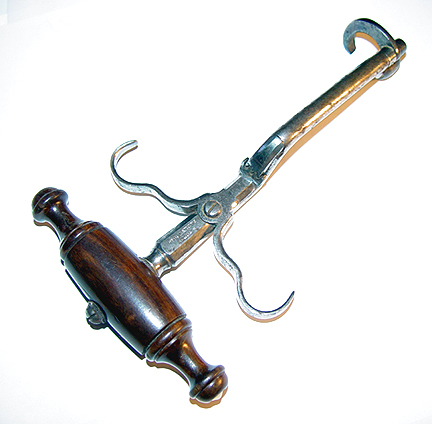The image depicts a metallic tool with a finely finished wooden handle, likely stained and varnished. The handle, located towards the base of the tool, is dark oak. Extending from the handle is a sleek metal shaft that culminates in a more intricate apparatus. This apparatus includes a central screw and two claw-like hooks on the sides, suggesting it might clamp onto or interact with another item. At the very end of this tool, there's a hook, and near the top, it features elements akin to a delicate hammer. The tool resembles a device that could be used for opening wine bottles, although its exact purpose remains uncertain. The entire object is displayed on a plain, white surface, providing no contextual clues about its size or specific use.